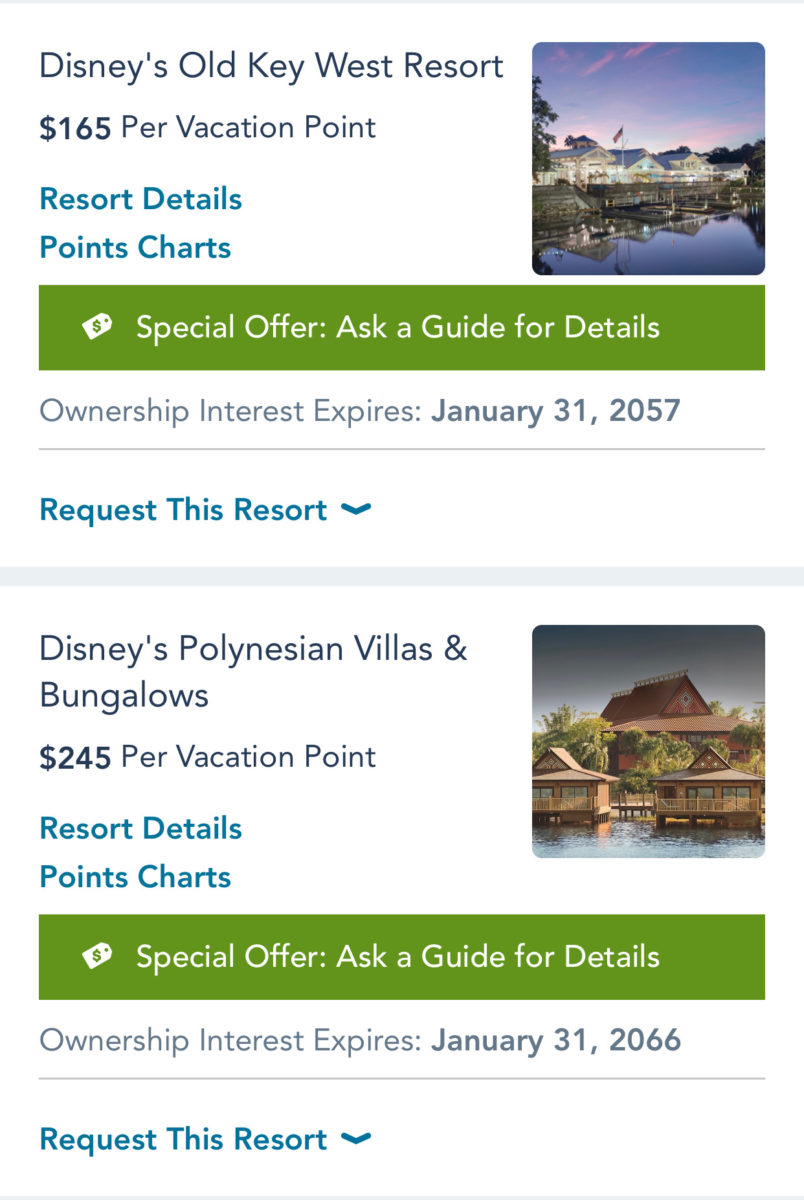The image showcases a webpage advertising Disney's Old Key West Resort and Disney's Polynesian Villas and Bungalows. The advertisement for Disney's Old Key West Resort highlights a special offer price of $165 per vacation point. The webpage includes clickable links for "Resort Details" and "Points Charts" which are presented in blue text. There is a green notification strip that mentions a special offer, encouraging viewers to "Ask a Guide for Details." Additionally, text informs that ownership interest for this resort expires on January 31, 2057. 

The image prominently features a stunning photograph of Disney's Old Key West Resort captured at sunset. The resort's structure is beautifully reflected in a serene body of water, with a sky transitioning to shades of pink and blue. Behind the resort, lush trees add to the picturesque scenery, with a notable tree situated on the left side of the frame.

Further down the webpage, the next section advertises Disney's Polynesian Villas and Bungalows at a rate of $245 per vacation point. Similar to the first section, there are clickable links for "Resort Details" and "Points Charts." A captivating photograph accompanies this listing, showcasing the Polynesian-style architecture with one larger building and two smaller overwater bungalows. Text in green reiterates the special offer, urging viewers to "Ask a Guide for Details," and ownership interest for this resort expires on January 31, 2066. This section also allows users to "Request This Resort," with a corresponding dropdown arrow for further options.